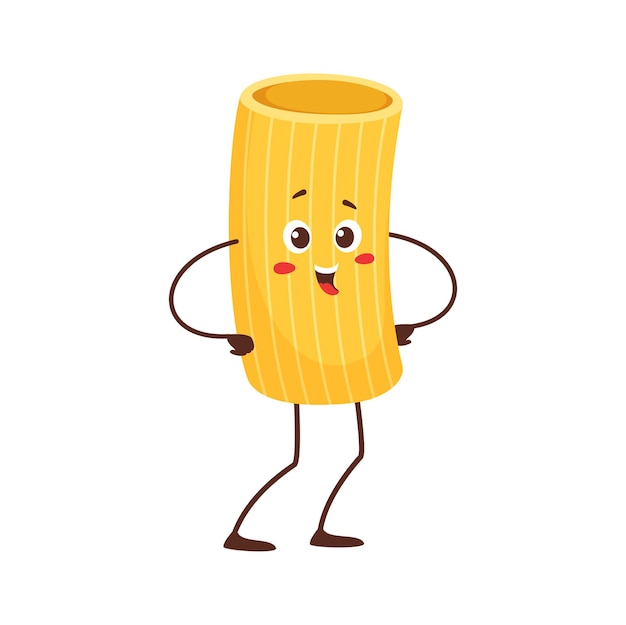This image is a stylized cartoon drawing of a piece of penne pasta, round and tubular with a yellowy-orange coloration accented by lighter vertical lines to suggest dimension. This humanized pasta character features expressive black and white eyes with brown eyebrows above, and red oval cheeks beneath. Its open, smiling mouth reveals a red tongue against a black background, and a white bar representing teeth. The character's very thin, semi-circular arms extend from its center and fold near its chest, while similarly skinny legs end in tiny feet, bent slightly at the knees. The overall appearance of this animated pasta character exudes a joyful, anthropomorphic charm.